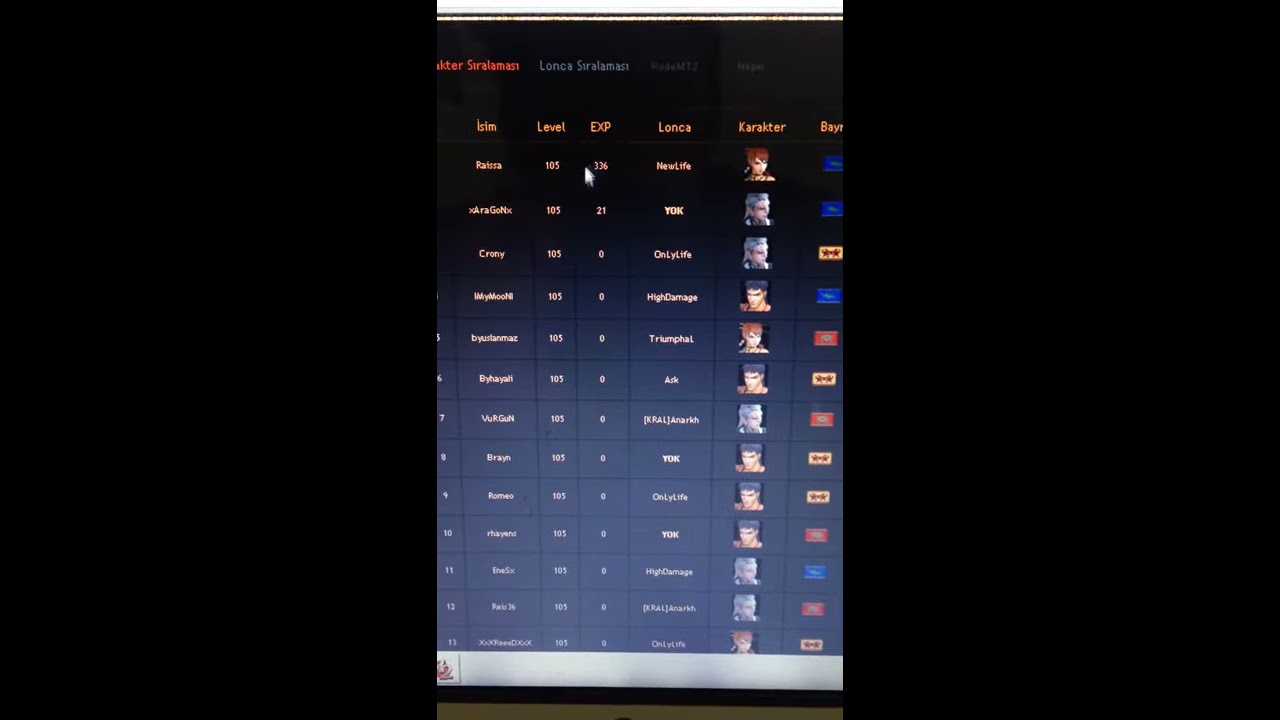This image is a screenshot of a digital device displaying a leaderboard from a video game or app game. The background features a gradient from black at the top fading into a lighter gray at the bottom. The leaderboard is organized into a grid with six vertical columns and 15 horizontal rows, listing various details about players.

Starting from the leftmost column, which contains text likely representing player names or unique identifiers, the text is in white and not uniform, making it indiscernible. The second column appears to be a numerical column with the heading "Level," indicating each player's level in the game. The third column also contains numerical data with an unclear heading, possibly related to experience points or scores. The fourth column, located centrally, again features white text that could denote player names. The fifth column includes square icons representing the avatars of the players. The final column on the right edge consists of differently colored squares and rectangles ranging from blue to yellow to red, although the specific purpose of this column is unclear. 

Throughout the columns, text such as "Cyralamast," "Lanka," "Reysa," "Zera," "Gonks," "Ai Maimou," "Baiuslanmaz," "Triumpha," "Baihali," "Virgun," "K-Rael," "Anark," "Brian," "Romeo," "Reigns," "NS," "X-Rael," and others are visible, along with numerical values such as "105," "336," and "21." The descriptive roles like "new life," "only life," and "high damage" are also noted, suggesting roles or statuses within the game. The bottom of the image features a white bar without any additional text or identifying features.

The overall style is distinctly digital and video game-oriented, characterized by a mix of bright and subdued colors including blue, dark blue, black, white, gray, brown, red, beige, yellow, and orange. The focal point is the vertical list of players and their corresponding information, with character images and detailed numerical data displayed prominently.